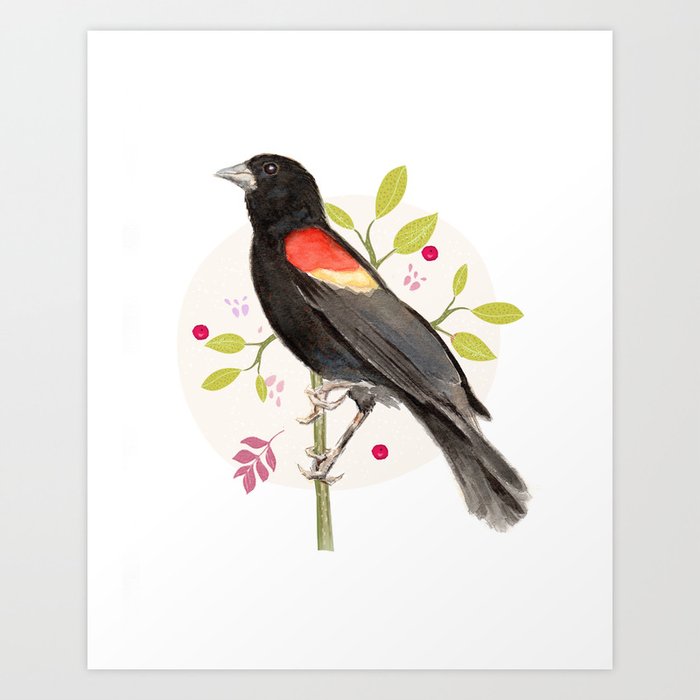The image is a detailed illustration, possibly a digital capture of a painting, depicting a red-winged blackbird. The bird is primarily black, featuring a striking red patch on its shoulder with an underlying yellow stripe that blends into the red, reminiscent of the Pepsi logo’s curve but in red and orange hues. It has a gray beak and a black eye. The bird is perched on an upright green stem with teardrop-shaped, bright lime green leaves. Scattered around the branch are three pieces of red fruit, positioned artistically without appearing to be directly connected. The backdrop is characterized by a light grey background with a white canvas or paper at the center. Enhancing the composition is a pale pink circle behind the bird, adding contrast. The painting also includes additional light pink leaves and various muted green berries, contributing to the overall aesthetic. The artist's brush strokes are subtly suggested, indicating the image may indeed be a painting.